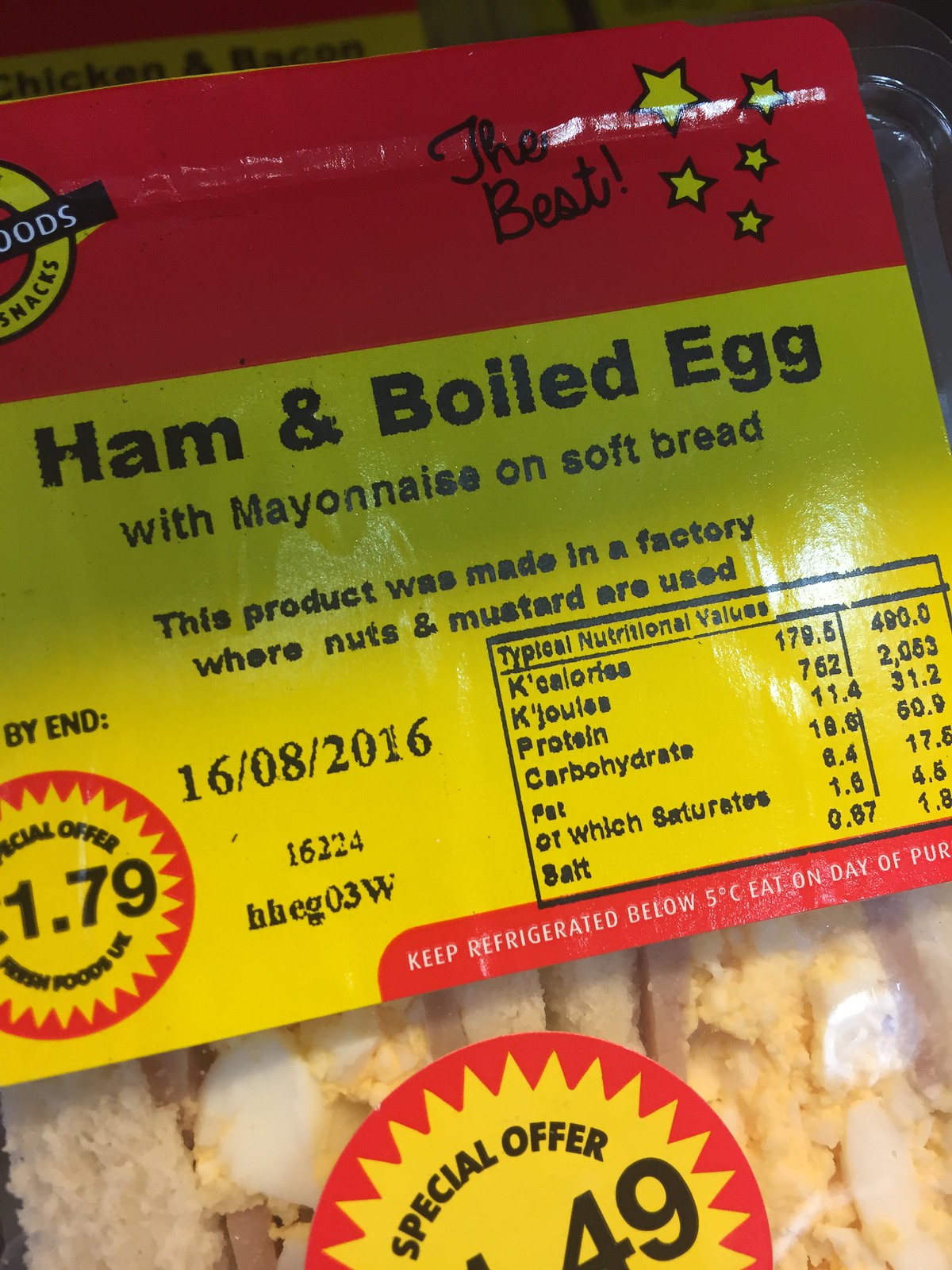The image showcases a close-up view of a food package labeled "Ham and Boiled Egg with Mayonnaise on Soft Bread." At the top of the packaging, there is a partial logo featuring a yellow ring with the letters "OODS" in white against a black background. Adjacent to this, the text "the best!" is written in black cursive, followed by five small yellow stars outlined in black—all set against a red background.

Below the logo, the product description is printed in black text: "Ham and Boiled Egg with Mayonnaise on Soft Bread. This product was made in a factory where nuts and mustard are used." The date "16-08-2016" is also present, indicating the production or expiration date.

A label announcing a "Special Offer: 1.79" is positioned prominently, alongside a black square that displays nutritional information. Another red label advises, "Keep refrigerated below 5 degrees Celsius. Eat on day of purchase." Through a clear plastic section, the contents of the package are visible, highlighting the ham and boiled egg filling. An additional sticker with a sun-shaped emoji and a red ring reinforces the "Special Offer" message.